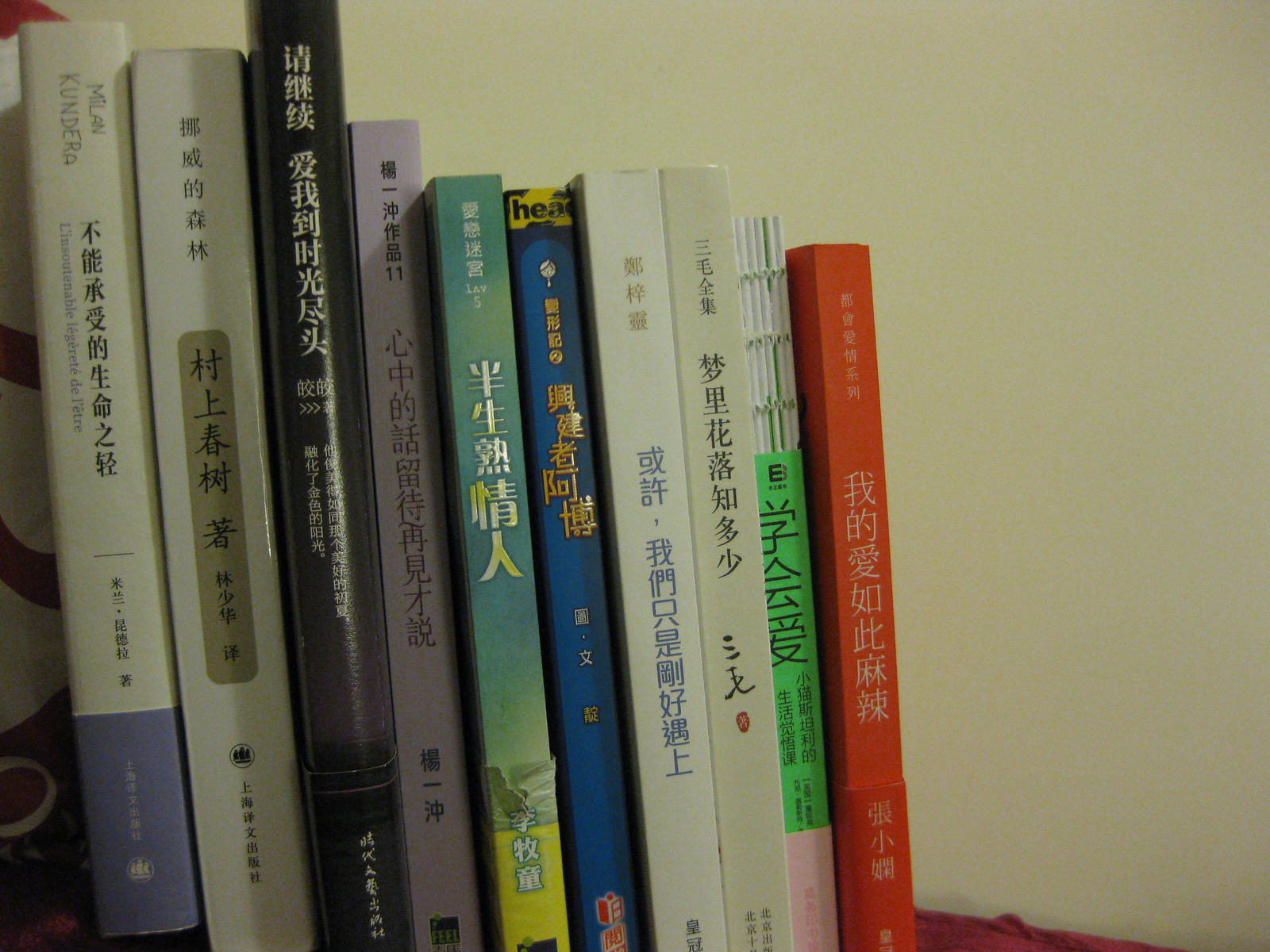In this indoor photograph, a series of ten vertically stacked books with Chinese or Japanese characters on their spines stand against an off-white, cream-colored wall, resembling a makeshift bookshelf. The books, arranged almost from tallest to shortest except for the third book, which is the tallest, have varied spine colors: the far-left book is white and purple; next is white and gold; then black and white; followed by black and purple; blue and yellow and green; yellow, blue, and gold; white, blue, and gold; black, white, and red; white, black, and green; and finally, red and white on the far right. These thin, possibly 50-page books include both hardcovers and softcovers, placed neatly in what might be a corner nook of someone's bedroom or home. The lower part of the image features some red fabric, adding a touch of color contrast to the scene.